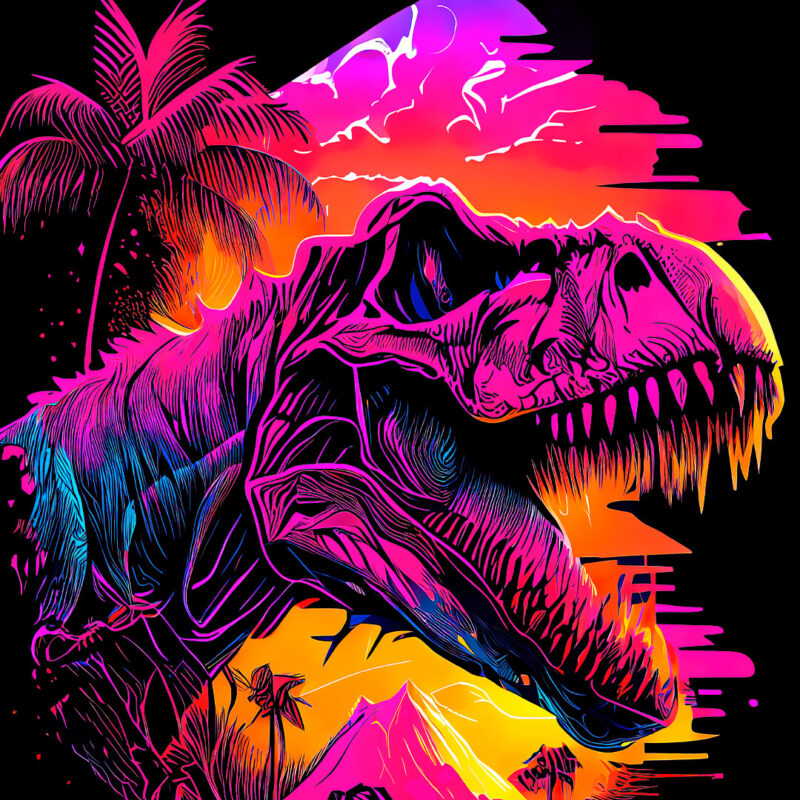This vibrant neon illustration vividly captures the essence of 1980s neon mall art. Dominated by electrifying hues of pink, orange, purple, and black, the central figure is a ferocious Tyrannosaurus rex. This T-Rex features gaping jaws displaying razor-sharp teeth, exuding an intimidating and menacing presence against a backdrop that radiates a sunset-like gradient of oranges and pinks. The intricate use of line work gives the T-Rex a fossilized appearance with finely detailed textures, reminiscent of pen and ink artistry, possibly with added felt texture for depth.

The T-Rex stands before a vivid sunset, further enhanced by bright oranges, pinks, and purples, as palm trees and mountainous landscapes, possibly even a volcano, adorn the scene. Highlights of blue within the dinosaur and fiery eyes add to the dramatic contrast against the pitch-black background. The entire composition appears poised to glow under a blacklight, suggesting an airbrushed design meant to captivate with its dazzling neon brilliance and meticulously detailed features.